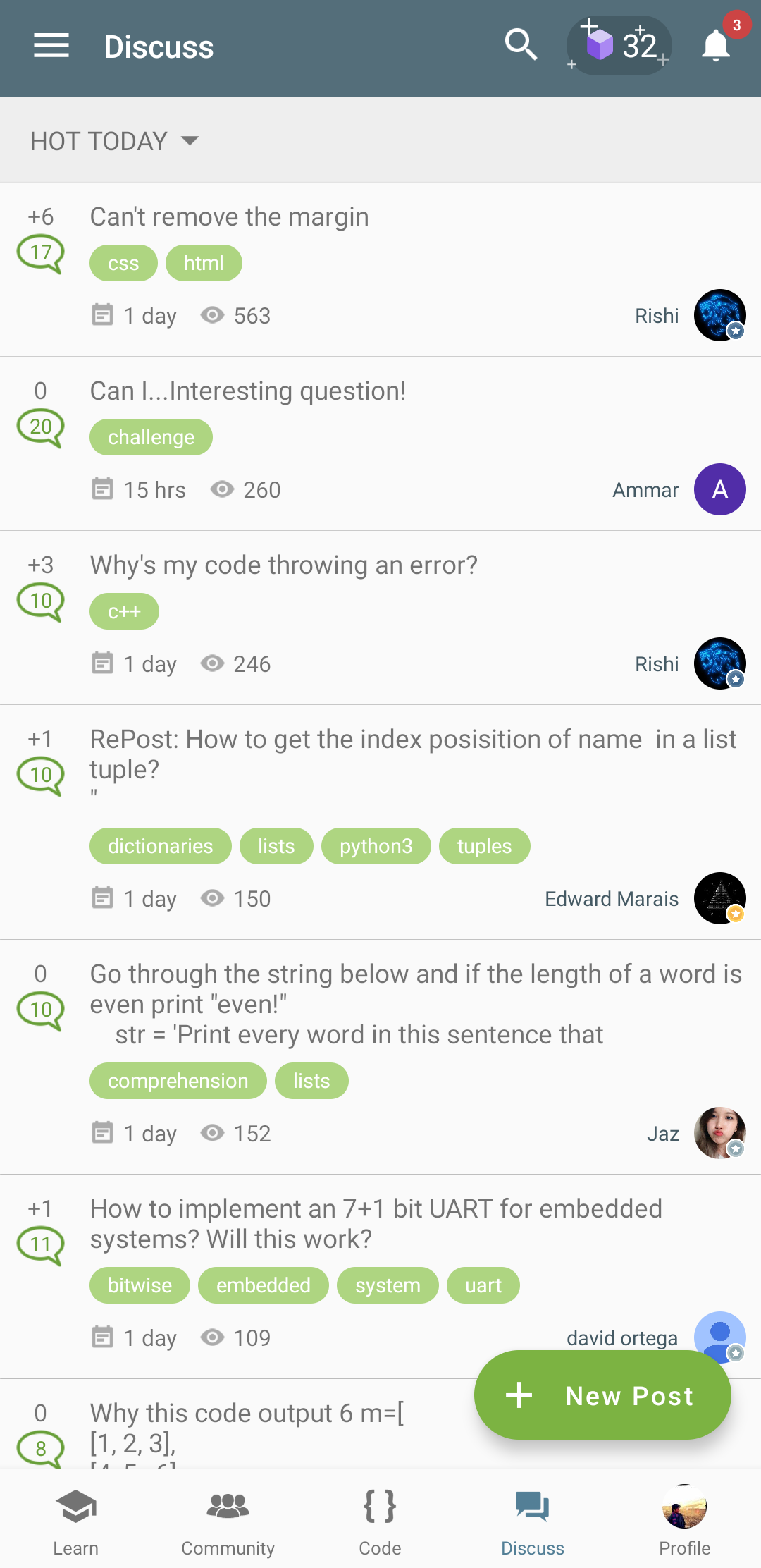This screenshot shows a mobile interface of a discussion board tailored for programmers. The layout is reminiscent of Reddit but isn't Reddit or Discord. At the top, there's a "Discuss" section prominently featuring trending topics labeled "Hot Today." Below this header, several discussion threads are visible, with topics such as "Can't remove the margin," "Can I ask?" "Interesting question," and "Why is my code throwing an error?" Each thread appears to attract considerable engagement, with around 50 responses per post, indicating an active and responsive community focused on solving programming-related issues and sharing information.